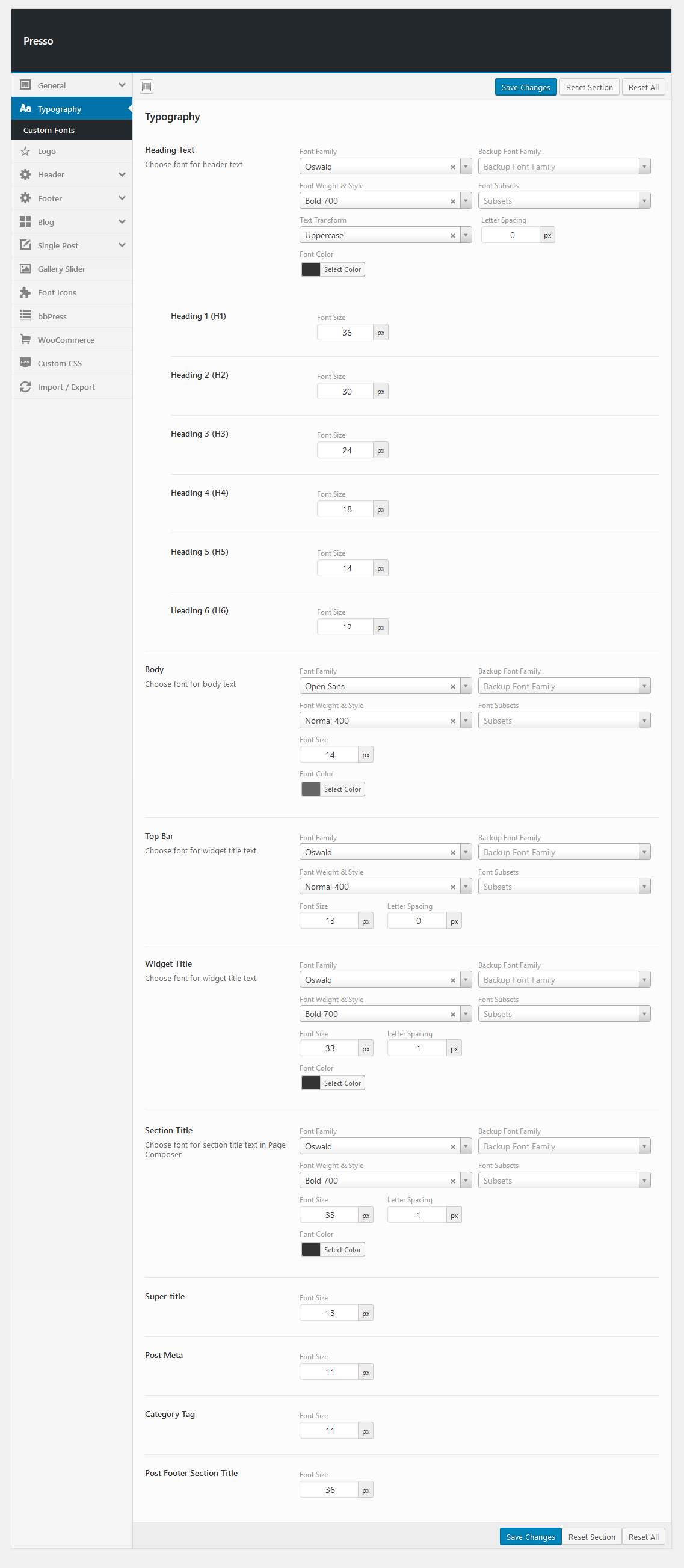**Detailed Caption:**

In this image, we see a comprehensive interface of a web-design tool being used to customize the typography of various elements on a webpage. The user is adjusting settings for different text components such as headers, footers, and blog posts. More specifically, the interface includes options for custom fonts and font icons, and displays features like the "Glory Slider," "BB Pers," and "WooCommerce" integration.

An extensive array of typography customization options is present. Users can import or export their settings and have the choice to save changes or reset sections. For the heading text, the user has chosen the "Oswald" font with a bold weight of 700 and set the text to transform to uppercase. There's also a backup font family option to ensure compatibility.

Further customization details show adjustments for the super title font size set to 13 pixels, post meta font size at 11 pixels, and category tag font size also at 11 pixels. The post footer section title has been set to a substantial 36 pixels in font size. Additionally, widget titles are being customized with the "Oswald" font family to maintain a cohesive design across the website.

This meticulous level of detail highlights the extensive customization capabilities offered by this web-design tool, catering to designers who seek precise control over their webpage's typography.